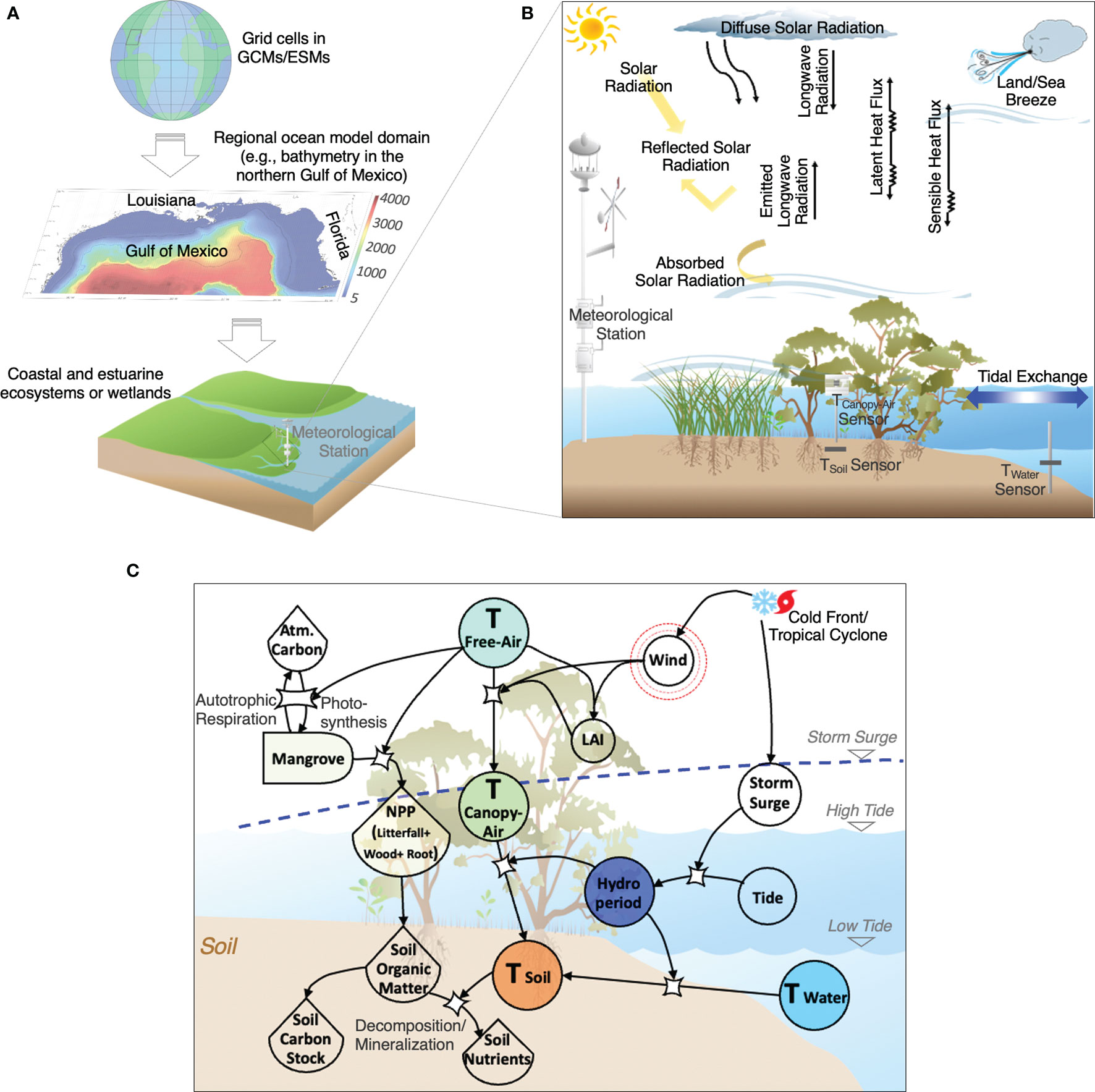The image is a detailed, scientific diagram divided into three sections labeled A, B, and C. 

Section A illustrates a global perspective with a picture of the world globe and detailed text indicating grid cells, GCMs (Global Climate Models), and ESMs (Earth System Models). This section also pinpoints Louisiana and the Gulf of Mexico, emphasizing their importance in a regional ocean model domain. There is a sub-diagram showcasing coastal and estuarine (Euphranian) ecosystems, depicted in different colors—red, green, and purple.

Section B delves into the mechanics of a meteorological station, focusing on diffusing solar radiation. It visually explains the interplay between land and sea breezes, and how solar radiation impacts these processes. The diagram includes the Sun, a body of water illustrating tidal exchanges, and the interaction between different components like the ocean floor, river, lake, and coastal vegetation.

Section C focuses on atmospheric conditions during a cold front or tropical cyclone. It features a chart illustrating the effects of these weather events on soil. This section includes various labeled circles connected by arrows, depicting the interrelations between aspects like wind, canopy air, and free air in scientific terms.